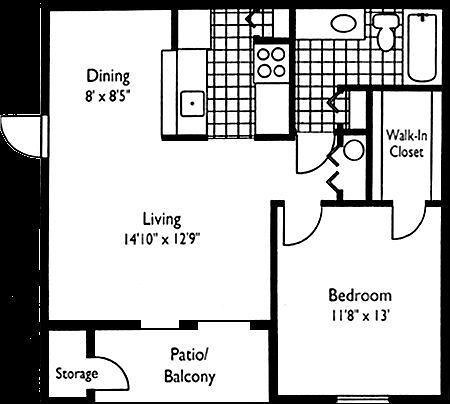The image displays a detailed black-and-white drawing of an apartment layout. The design features a square architectural blueprint comprising several labeled areas. The dining area, denoted as "Dining," measures 8 by 8.5 feet and is situated adjacent to a spacious living room labeled "Living," which is 14.10 by 12.9 feet. A generously sized bedroom, labeled "Bedroom," measures 11.8 by 13 feet and includes a walk-in closet for added storage. The kitchen area is conveniently located beside the dining area. The bathroom is well-appointed with a bathtub, shower, wash hand basin, and toilet. Additionally, the layout includes a patio and extra storage space, enhancing the apartment's functionality and comfort.